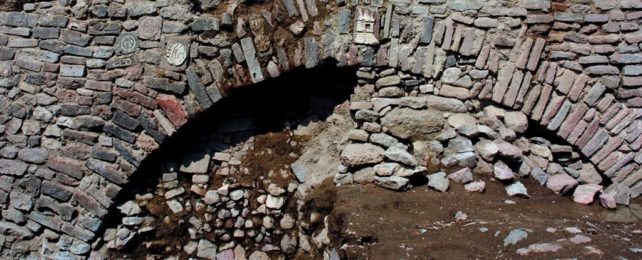The image depicts an outdoor setting featuring the base structure of what appears to be a stone bridge or possibly a man-made cave. The focal point is a stone archway, partially obstructed by a stack of rocks on one side while the other side remains open. This archway is constructed from various shades of cemented stones, including gray, red, brown, and even some blue hues, all set on a foundation of moist, brown dirt. The partially blocked opening creates a dark shadow within the arch, adding to the impression of a tunnel or cave entrance. Although not much else is present in the image, the intricate arrangement of stones forming the arch hints at its historical or structural significance. The overall ambiance suggests an aged, somewhat eroded structure with a mysterious, darkened interior.